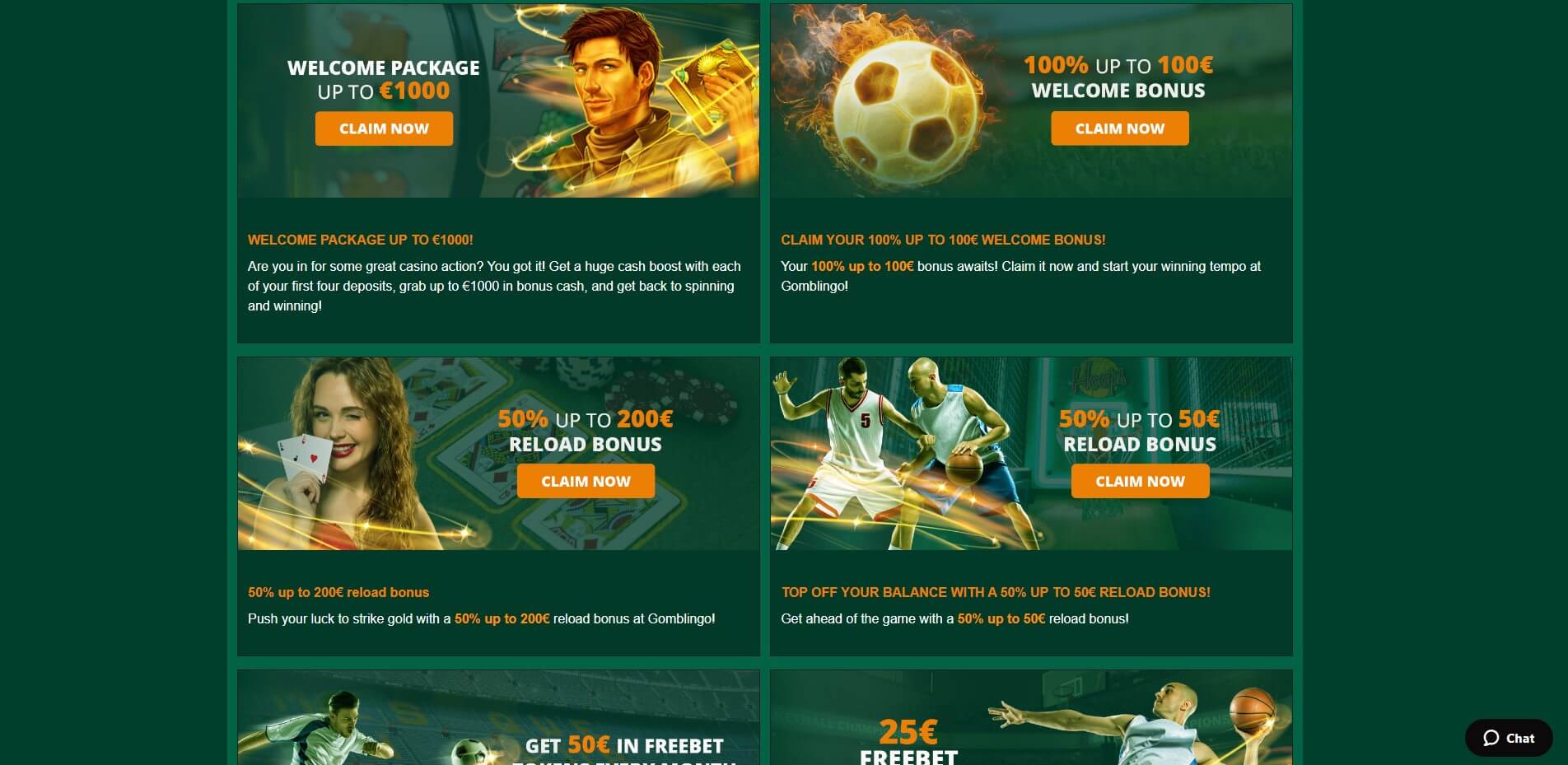The image showcases a vibrant website interface with a teal background, featuring various promotional game thumbnails arranged in a grid within a highlighted box. 

**Top Left Thumbnail:**
A promotional image for a welcome package offering up to £1,000, depicted with a man holding a book. The text reads, "Welcome package up to £1,000. Claim now."

**Top Middle Thumbnail:**
An exciting graphic of a soccer ball enveloped in flames, promoting a 100% welcome bonus up to £100. The accompanying text states, "100% up to £100 welcome bonus. Claim now."

**Bottom Left Thumbnail (Middle of Page):**
An engaging visual of a woman with long, wavy brown hair and red lipstick, winking while holding two cards—a visible Ace of Hearts and an Ace of Spades—close to her face. The promotion next to her offers a 50% reload bonus up to £200, with the words, "50% up to £200 reload bonus. Claim now."

**Bottom Right Thumbnail (Middle of Page):**
A dynamic image of two basketball players in the heat of the game. The player on the left has pale skin, dark hair, a dark goatee, and wears a white jersey with red trim and the number 5, paired with white shorts with red trim. He has one arm extended to block the other player, who has a darker complexion, a bald head, a white jersey, and blue shorts. This player is in possession of the ball, and the text beside the image reads, "50% up to £50 reload bonus. Claim now."

**Bottom Thumbnails:**
Two additional thumbnail images are partially visible below the main thumbnails, cut off at the bottom edge, leaving their contents obscured. 

Overall, the website layout effectively highlights various gaming promotions, each with distinctive and engaging visuals to attract users.